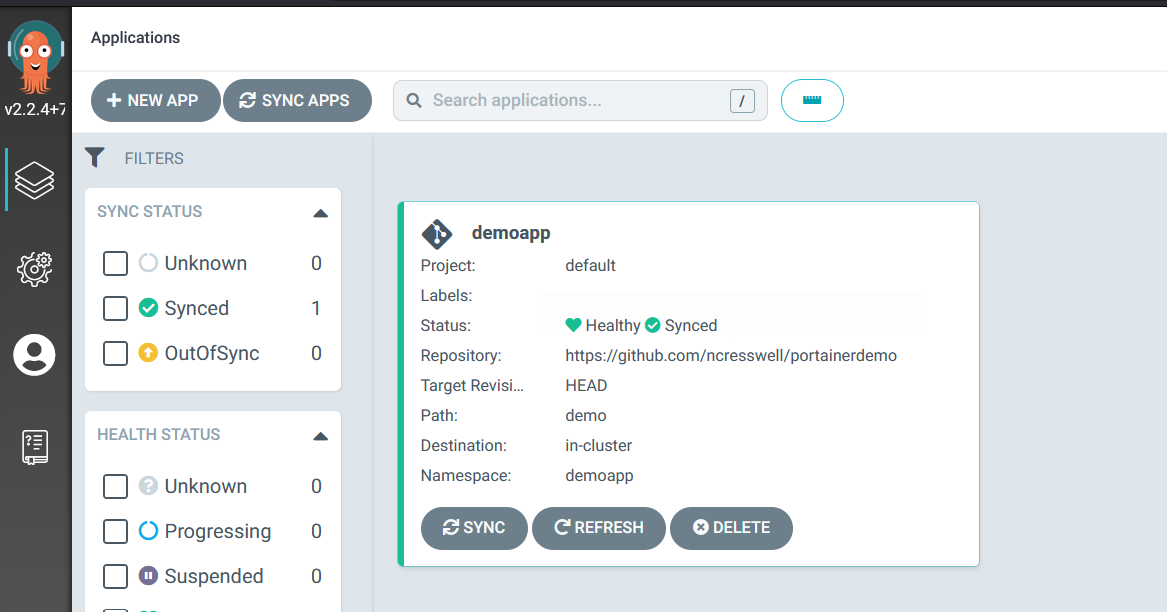This image showcases a user interface of a software development platform, likely a web-based application designed for managing projects. The right half of the screen is dominated by a section labeled "Demo App" and includes details such as project status, default settings, and a list of various items. There's a mention of "Compository" and "GitHub," indicating that this interface is related to programming and code repositories.

On the left side of the image, there is a navigation bar with several filters—sync status, health status, and others—probably utilized for organizing and tracking the progress of different files within the project. Notably, there is an image of a happy, cartoonish squid-like creature wearing a translucent astronaut helmet, which is associated with the version number 2.2.4+7. This might be the mascot or logo for the software or a particular feature within it.

Additionally, the interface includes functional buttons such as "Sync Apps" and "New App" at the top, indicating options for synchronizing applications or creating new projects. The overall look suggests a comprehensive tool for developers to manage their work with detailed oversight and organization.